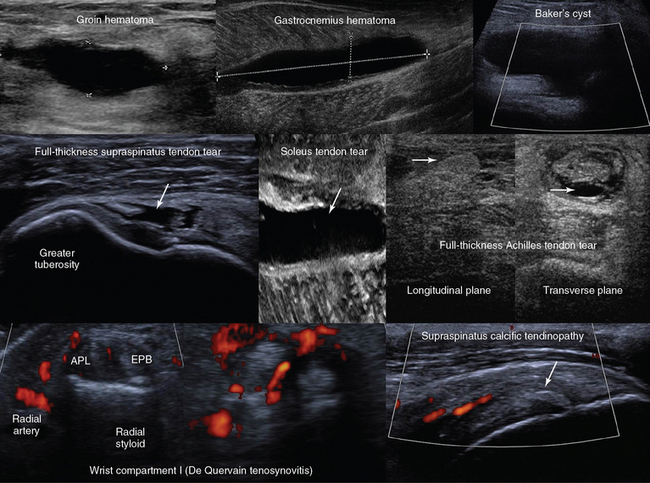This combined photograph features nine detailed radiological and high-imaging x-rays, illustrating various medical conditions predominantly through transverse and longitudinal plane scans. The images, often labeled with complex medical terminology, suggest different types of soft tissue injuries and abnormalities within the human body. Starting from the top left, the labeled scans depict a groin hematoma followed by a gastrocnemius hematoma in the top middle. To the top right, there's an image identifying a Baker's cyst. Moving to the middle row from left to right, there is a full-thickness supraspinatus tendon tear indicating greater tuberosity, followed by a soleus tendon tear, and subsequently a full-thickness Achilles tendon tear. The bottom section exhibits a radial artery with related labels such as APL, EPB, and radial styloid, highlighting areas like the wrist compartment and de Quervain tenosynovitis. Additionally, noticeable are vividly colored regions in reddish-orange indicating possibly inflamed or damaged tissues. Completing the array, the bottom right scan shows supraspinatus calcific tendinopathy. The precise annotations and visual emphasis on tears, cysts, and hematomas make this a highly specialized series of diagnostic images, likely intended for professional evaluation and understanding.